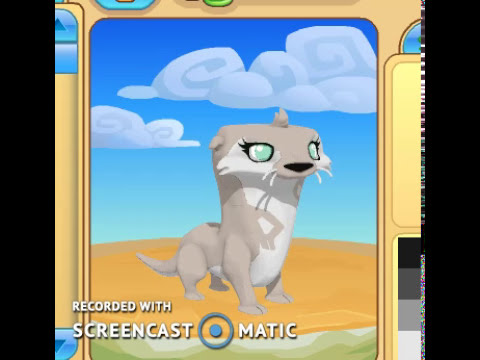The image is a digitally created, rectangular, horizontal cartoon with black borders on the left and right sides. It's a screen grab from a video made with Screencast-O-Matic, clearly indicated by the white text at the bottom that reads "recorded with Screencast-O-Matic." The "O" in Screencast-O-Matic is depicted as a large white circle with a small frame inside containing a solid blue circle, resembling a video recording button.

The scene portrays a whimsical landscape with brown, sandy ground at the bottom, and a vibrant blue sky accented by fluffy white clouds. Dominating the scene is a peculiar, grayish creature that stands on four legs. Its appearance is an odd blend, somewhat reminiscent of a cat but with a grotesquely shaped catfish-like face, featuring a long, thick neck, blue eyes, a tuft of hair on top, and whiskers jutting out from either side of its mouth. The creature's body is white in the front and has tan sides, further highlighting its unique and fictional nature. The overall atmosphere of the image is enhanced by an additional yellow frame, adding to the cartoonish and playful theme.